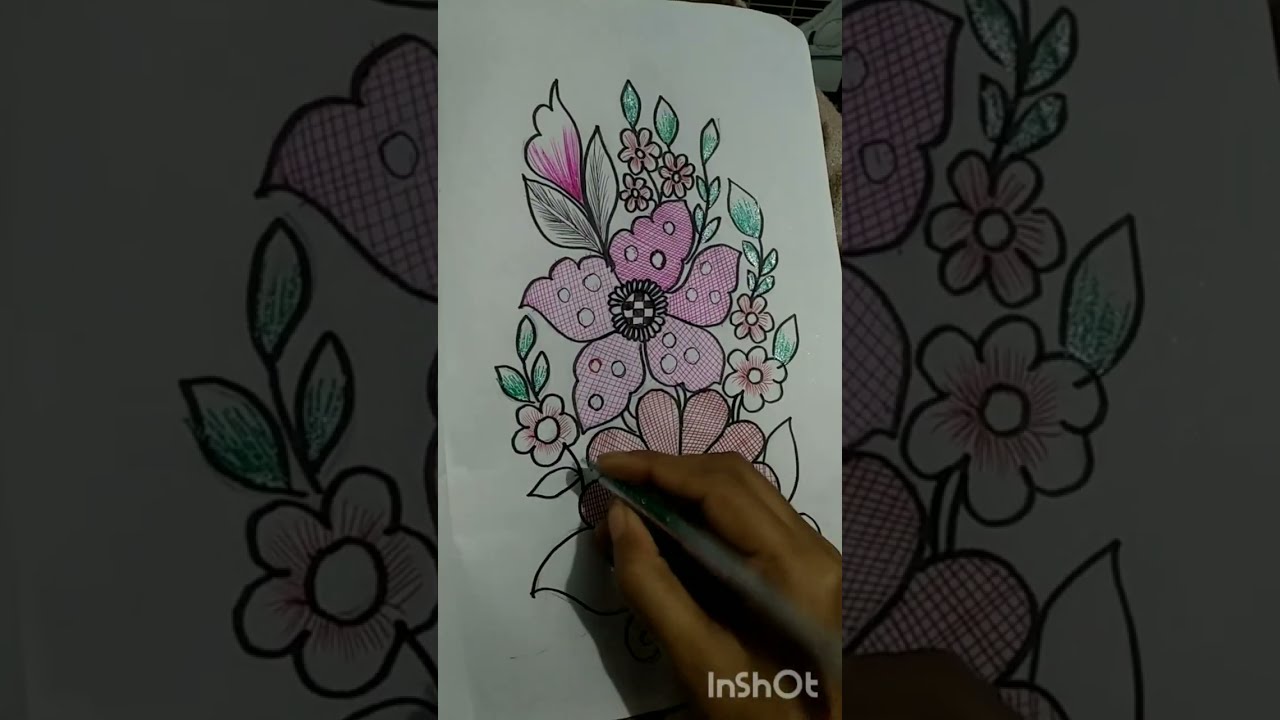The image is a striking composite featuring two contrasting states of exposure. The background is a dark, blurred underexposed sketch of flowers and leaves, drawn in black ink on a white sheet, creating a dim, almost ethereal backdrop. Superimposed on this background, occupying the central third of the vertical axis, is a sharply focused, normally exposed photo. This foreground image showcases a hand with medium dark skin, holding a gray pen, actively drawing on a similar floral sketch. The flowers and leaves are outlined in black and partially filled with vibrant red and green hues, employing hatching techniques for shading rather than complete coloring. Near the bottom of the foreground, the text "IN SHOT" is visibly printed in capital letters. The dual exposure enhances the artistic depth, highlighting the meticulous process of creation amid contrasting light conditions.